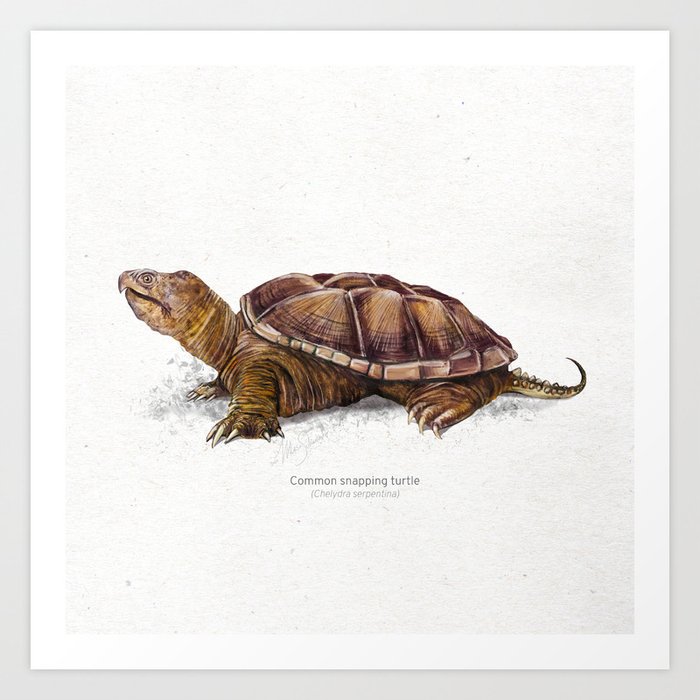The image is a detailed color illustration of a Common Snapping Turtle in a square format, set against a light gray background with a white border and a gray border around the edge. The turtle is brown and depicted in a left-facing profile. It has a large head with a pointed nose curving down over its lower lip, rounded eyes facing the viewer, and an overbite. The head is sticking upright from the shell, slightly higher than the shell. The turtle's body and four short legs are brown and wrinkled, each ending in claws. The turtle's flattish, dark brown shell has lighter brown raised portions with grooves in between the sections and a pinkish perimeter with vertically arranged segments and a horizontal band around the edge. The tail, thin and curved, is visible on the right side of the image. Underneath the turtle, black text reads "Common Snapping Turtle" with the Latin genus name in gray text in parentheses underneath.